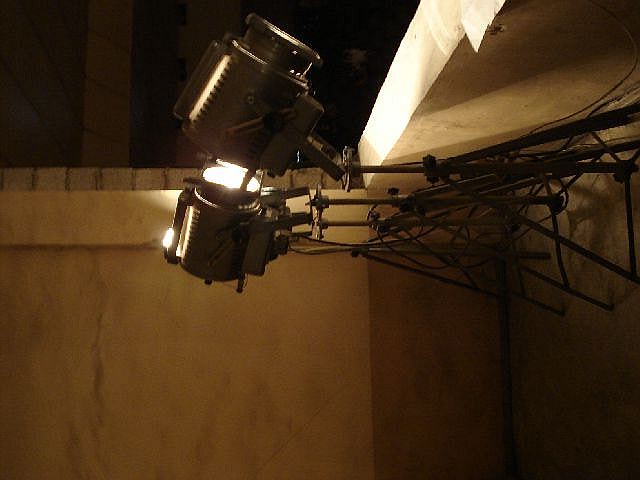The image features two adjustable spotlights, reminiscent of stage or theater lighting, mounted on a brown and beige wall with black metal supports. These spotlights are attached to triangular metal struts and are extending horizontally from the wall. The lights are connected to an external power source with several electrical cables, but we don’t see the actual lenses of the spotlights. The illumination from one spotlight is shining onto the wall and partially onto the other light. The background consists of brown and beige tones, with a darker section towards the top and a concrete border, possibly supported by a vertical 4x4 beam. The scene appears devoid of any text or markings, and the lights do not seem to be at full brightness, suggesting they may be remotely controlled. The orientation of the photo hints at the lights possibly being used in a venue setting, such as above a stage.